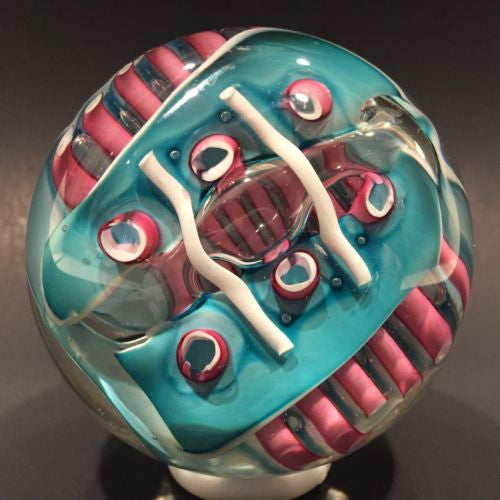This image captures a striking digital photograph of a glass sculpture that rests on a white-colored platform. The sculpture, shaped like a round bubble, showcases intricate, magnified interior textures that can be seen through its clear outer shell. Pink and blue mixtures converge inside the glass, creating abstract designs that don't form any distinguishable shapes but appear thoughtfully arranged. Near the top of the sculpture, there are six holes encircled by pink, with two white strips stretching across the surface. These strips partially obscure the pink and blue interior elements. Shiny and reflective, the sculpture features five long pink cords with white segments nestled under the object, enhanced by a blue backing. The scene includes a table supporting this captivating artwork, which is set against a grayscale and blue palette, leaving viewers to marvel at its complex, glass-encased beauty.